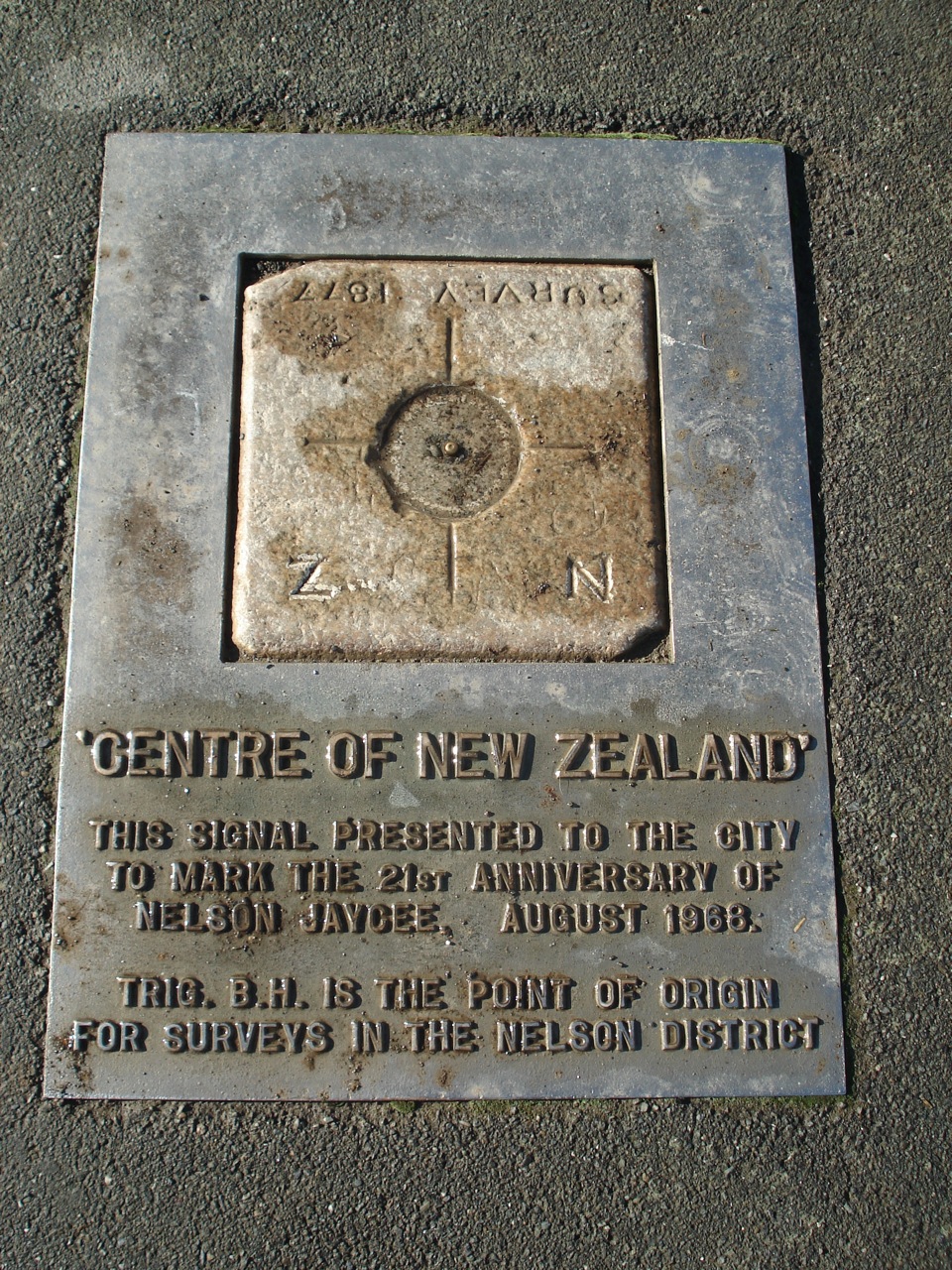The image is a vertically aligned rectangular photograph depicting a weathered stone plaque embedded in the ground, surrounded by gray and grainy cement. The stone, which appears gray with brown and weathered textures, features a central square section with a compass design. The compass shows lines pointing in cardinal directions and the text "Survey 1877" upside down at the top, with the letters "Z" and "N" carved into the left and right corners, respectively.

Around this central stone, there is a metal frame, likely stainless steel, inscribed with detailed information. The bottom section of the plaque reads, "Center of New Zealand, this signal presented to the city to mark the 21st anniversary of Nelson J.C., August 1968. Trig BH is the point of origin for surveys in the Nelson District."

Overall, the image effectively captures the historic significance of this survey marker, symbolizing its role as the trigonometrical point of origin for surveys in the Nelson District.